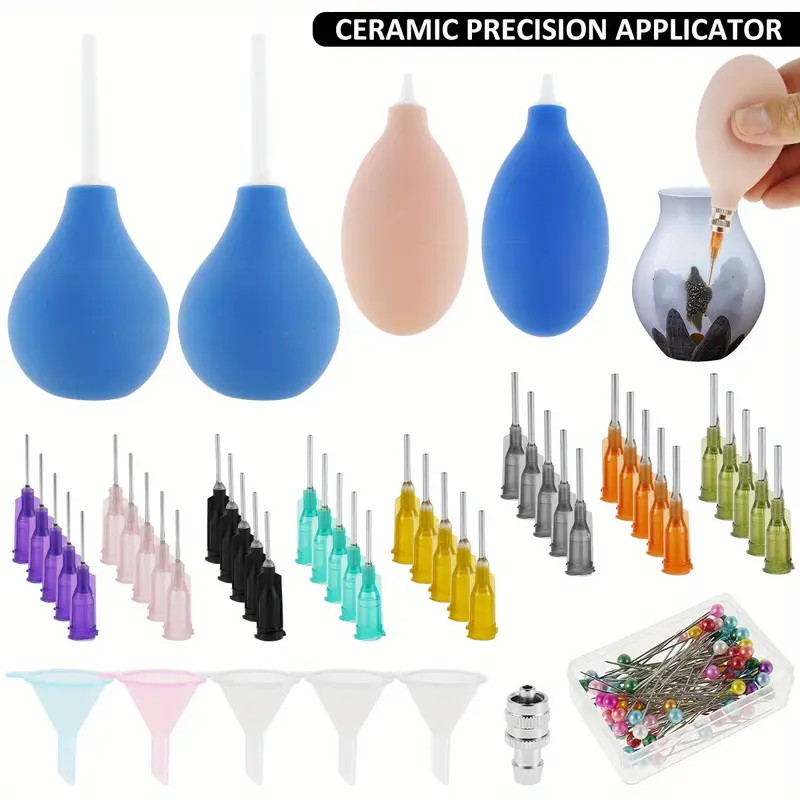This is a detailed photograph showcasing a variety of ceramic precision applicators and their tips. At the top, four applicators are arranged in a row: two with long blue stems, followed by one pink and one blue with shorter stems. On the right, an individual's fingers are shown using a pink applicator with a bronze tip to dispense black liquid into a small gray ceramic jar. Below this, numerous applicator tips are displayed in organized rows, color-coded as follows: purple, pink, black, teal, yellow, gray, orange, and green. Additionally, various funnels—including blue, red, and three white ones—are situated at the bottom left, accompanied by a metal tool, and a clear case containing round-headed straight pins with assorted colored tops can be found in the bottom right corner.